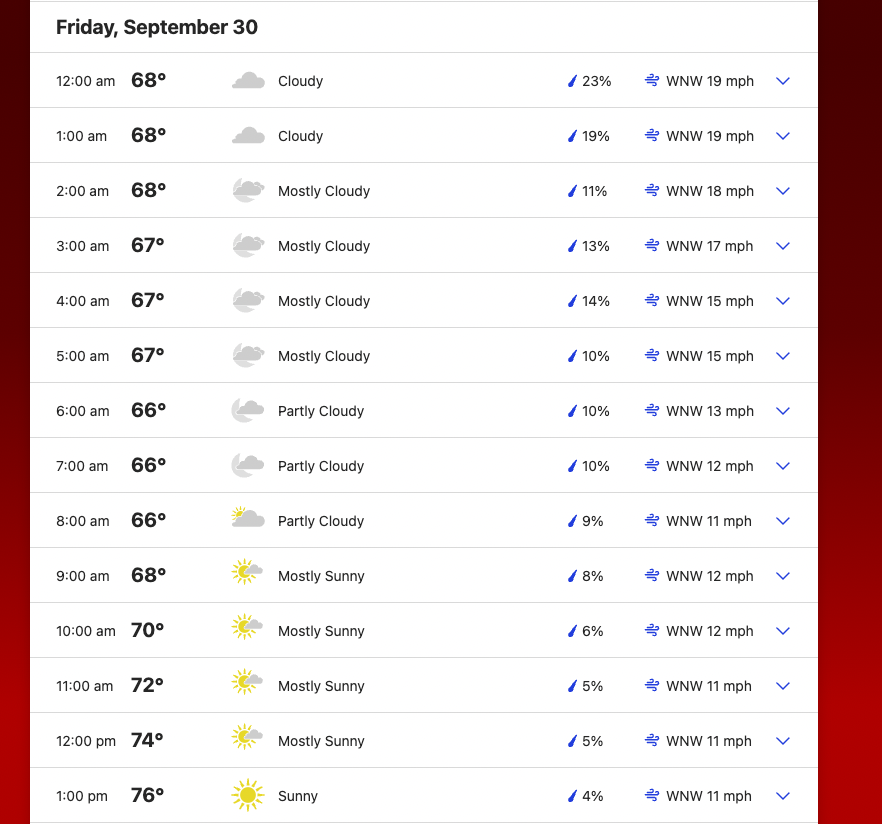The image is a screenshot depicting the upcoming weather forecast. On the left side, a gradient bar displays temperature changes, transitioning from dark red at the top, tapering into a slightly brighter red by the midpoint. The right side of the screenshot spans twice the width of the left side and features a gray line running horizontally across the top. Bold black text beneath this line reads "Friday, September 30th." Below this, each hour from 12 a.m. to 1 p.m. is detailed in a tabular format.

Each row includes:
- The time of day on the left.
- The corresponding temperature in bold and colored text.
- Weather conditions (e.g., cloudy, sunny, mostly cloudy).
- A percentage indicating the chance of rain.
- Wind speed and direction, represented with blue icons.

The hourly temperatures are as follows: 
- 12 a.m. to 2 a.m.: 68°F
- 3 a.m. to 5 a.m.: 67°F
- 6 a.m. to 7 a.m.: 66°F
- 8 a.m.: 68°F
- 9 a.m.: 70°F
- 10 a.m.: 72°F
- 11 a.m.: 74°F
- 12 p.m. to 1 p.m.: 76°F

A blue drop-down tab is located on the right side of each section for additional details. The forecast clearly distinguishes temperature variations, weather conditions, and chances of precipitation, providing a comprehensive hourly breakdown for planning the day ahead.